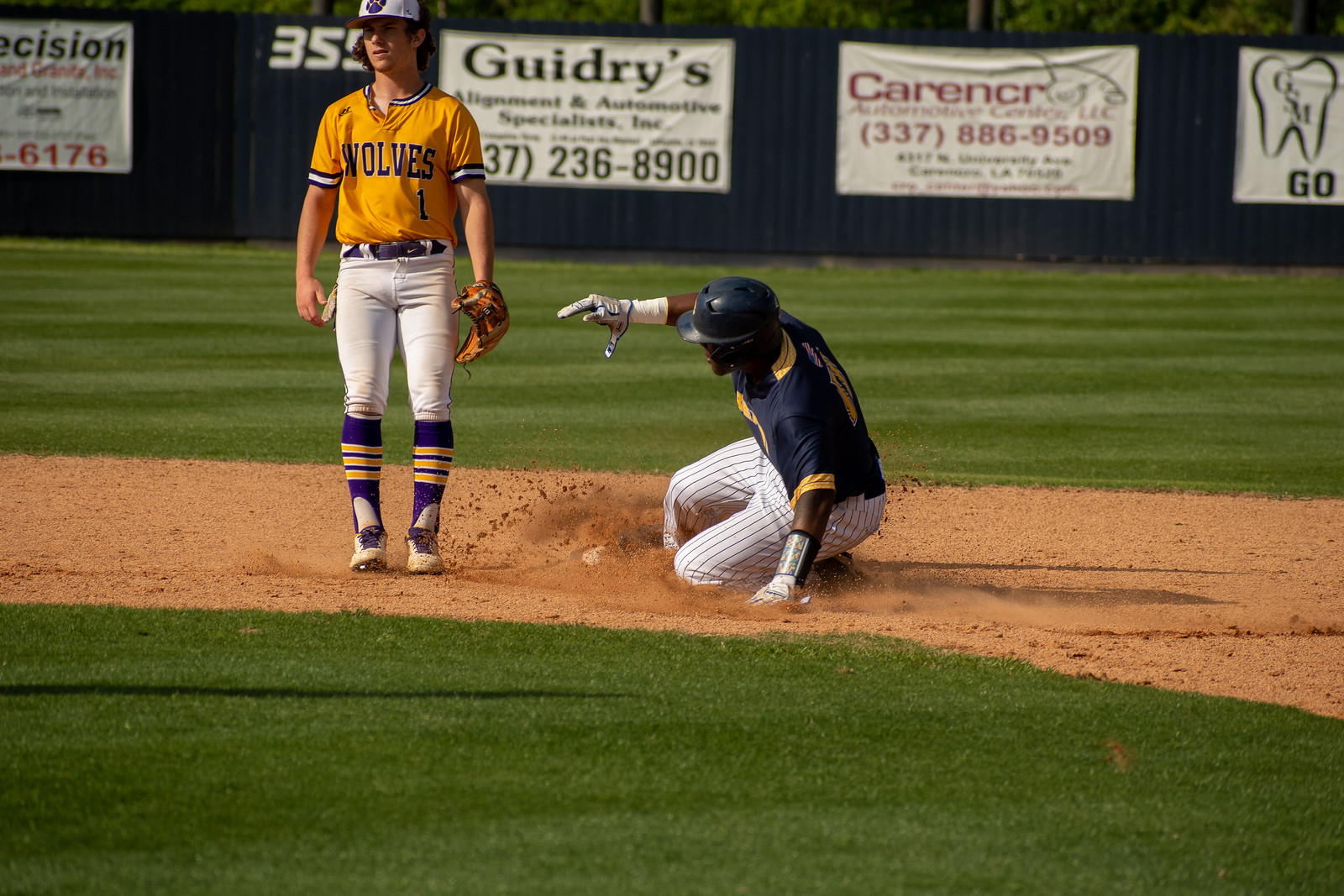This detailed image captures an intense moment during a daytime baseball game on a well-manicured, predominantly green field with freshly cut grass. At the center, a player wearing white pinstripe pants, a blue jersey with gold lettering, and a blue helmet, appears to be an African American man, slides into a base. The sliding action is directed towards another player from the opposing team, who is poised with a baseball mitt. This opponent is dressed in a distinctive uniform featuring a yellow jersey with purple and white stripes, and the word "Wolves" is emblazoned on it. He also sports knee-high purple socks, cleats, and a white cap with a logo. The infield area around them transitions from green grass to a brown clay-like dirt surface, common in baseball fields. Further into the background, an outfield wall adorned with advertisements from Gwydrize, Carencer, and Precision is visible, providing a spectrum of colors including green, tan, yellow, purple, white, red, and black. This lively, outdoor game scene is beautifully lit by natural daylight, capturing the dynamic movements and vivid colors of the players in action.